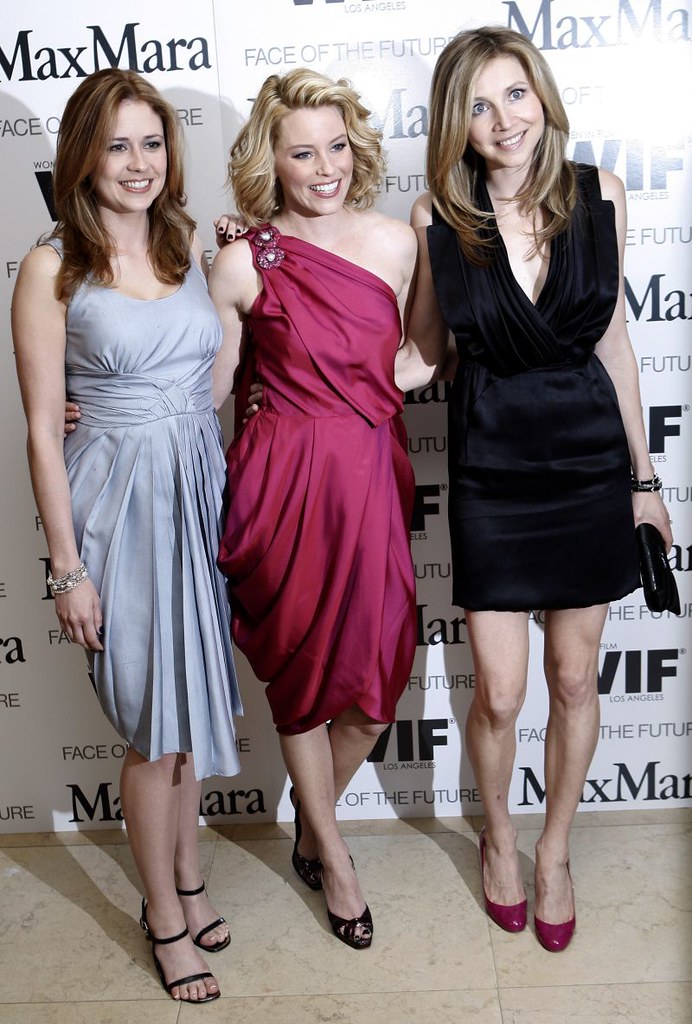The three women, all recognized as well-known movie or TV stars, are posing for a photograph in front of a white backdrop adorned with multiple repeated logos including "Max Mara," "Face of the Future," "WIF," and "Los Angeles," all in black text. They stand on a tan tiled floor, with the wall behind them taking up the top three-fourths of the image. On the left is the woman who plays Pam in "The Office," wearing black high-heeled sandals and a sleeveless purple dress, accessorized with a beaded wristband. In the center, another woman with blonde hair is dressed in a one-strap burgundy dress and black high heels, and she is holding a clutch in her left hand. To the right is a woman in purple high heels and a sleeveless black cocktail dress with a low neckline. Their attire features a mix of black, purple, and burgundy hues, while their fair skin and varying hairstyles add to the stylish, sophisticated atmosphere of what appears to be a high-profile event.